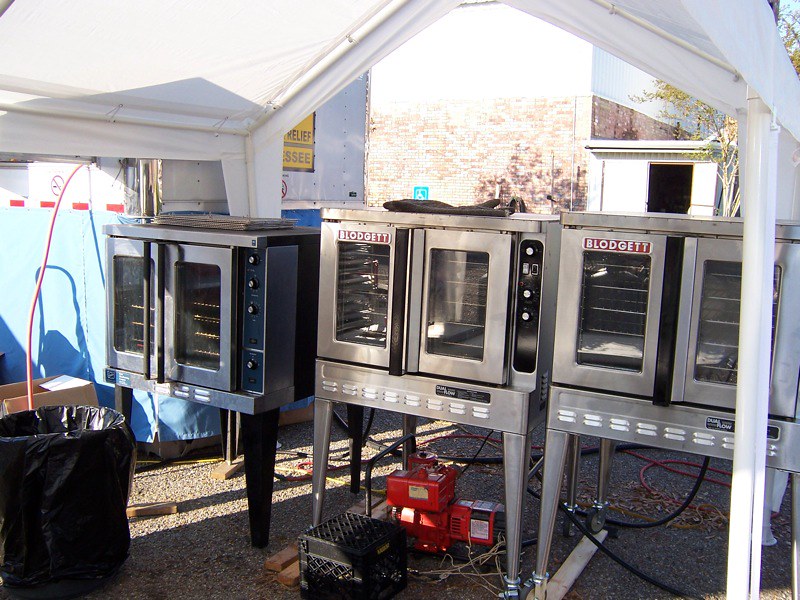This horizontal rectangular photograph captures an outdoor scene featuring three professional cooking ovens, likely Blodgett models, under a white tent canopy. The ovens, which are double-door and stainless steel, stand on four legs. The first oven has black legs, while the other two have silver legs. The second and third ovens bear the Blodgett label on the upper left corner of their doors—a red oval with the brand's name in silver lettering. 

Situated among cords and equipment, the middle oven has dials on its right-hand side. Underneath this oven, a red generator is visible alongside a black milk crate and a red extension cord coiled in a cardboard box. A blue tarp lies to the left of the setup, and a trash can with a black trash bag sits in the lower left corner of the frame, fully covering the can. 

In the background, there's a brick wall with a white building displaying a partially visible yellow sign that reads "RELIEF" and part of another word, "E-S-S-E-E." A tree is apparent in the upper right, casting its shadow on the scene, and a section of a handicapped parking space is visible beside the setup. A white pole runs nearly along the right edge of the frame, and the top portion of a triangular white roof or canopy is cut off at the top edge of the picture.